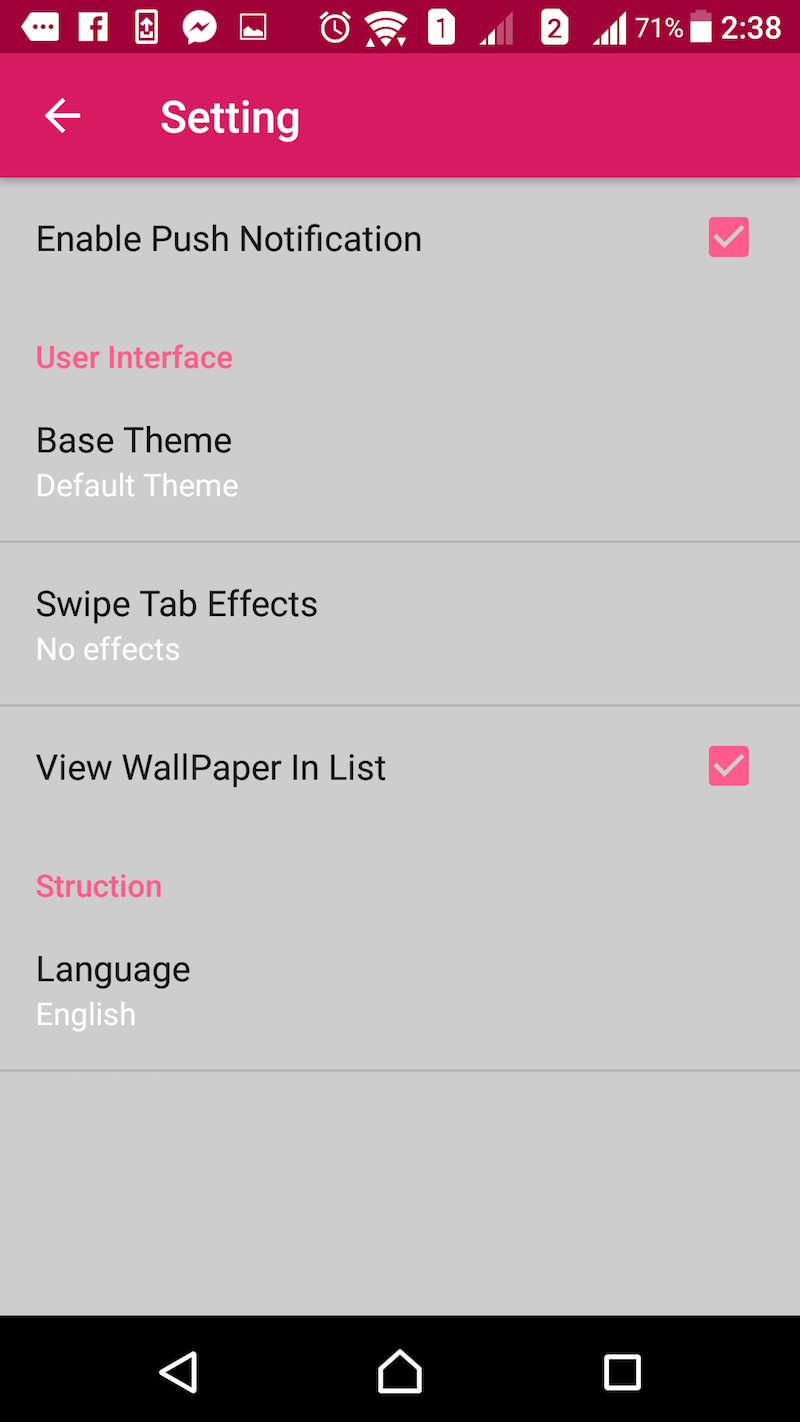Screenshot of a settings menu showcasing various customization options. The menu displays a variety of settings including "Enable Push Notifications", "User Interface", "Default Theme", "Swipe Tab Effects", "View Wallpaper and List", and "Language: English". The image appears to be illustrating a user navigating the settings to personalize their interface. The options for "Base Theme", "Default Theme", and "Swipe Tab Effects" are highlighted, along with repeated mentions of "User Interface", "View Wallpaper and List", and "Language", emphasizing the user's actions as they explore these settings.